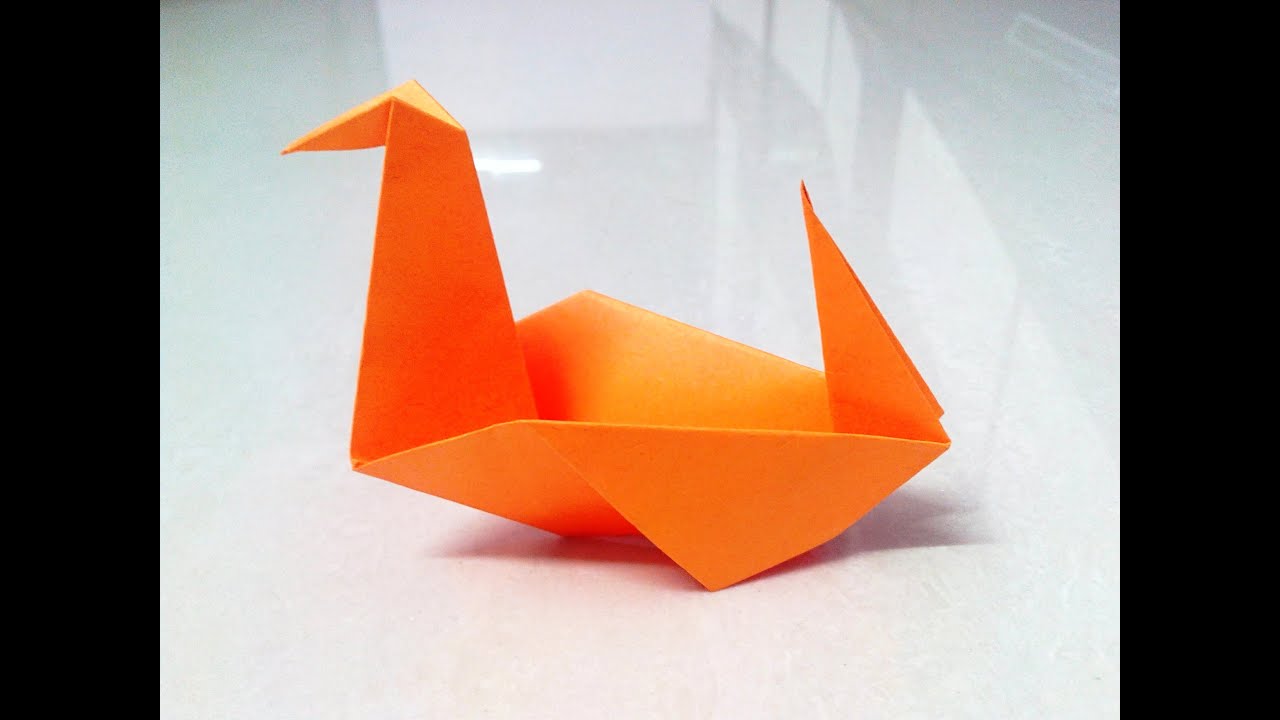The photograph showcases a meticulously crafted orange origami swan, captured up close and set against a pristine, glossy white background. The swan's smooth, crisp folds are highlighted by the light shining down from above, creating a delicate play of shadows and a clear depiction of the bright orange hues. The swan features a long neck with a sharp beak, a vertically folded tail, and wings angled downward, embodying the classic origami design. Two black rectangles on the left and right sides of the image frame the scene, further drawing attention to the origami figure. The background, slightly reflective, hints at faint, indiscernible shapes that add to the photograph's depth without distracting from the primary subject. This simple yet elegant piece of traditional origami stands out beautifully in the expertly lit and composed image.